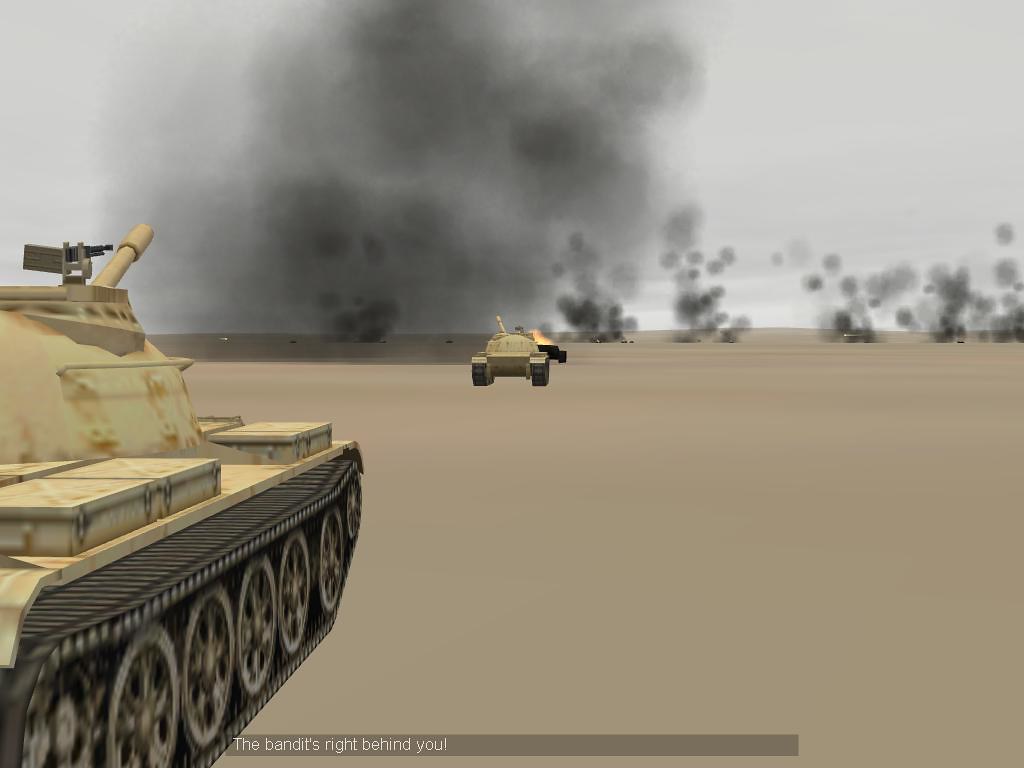The image is a detailed still from a video game, most likely from an older platform such as a PlayStation 2, PlayStation 3, or an Xbox. The scene is set in a desert-like environment with tan, sandy ground extending to the horizon. In the foreground, there are two large, khaki green and brown military tanks. The first tank is positioned slightly to the right with only its front half visible. The second tank is further ahead, and a black, charred vehicle that seems to be on fire lies in front of them. The scene is punctuated by dramatic black and gray smoke clouds, indicating ongoing explosions. The sky above is gray and featureless, enhancing the desolate atmosphere. At the bottom of the image, there's a black text bar that reads, "The bandits right behind you," adding to the sense of urgency and danger in the scene.